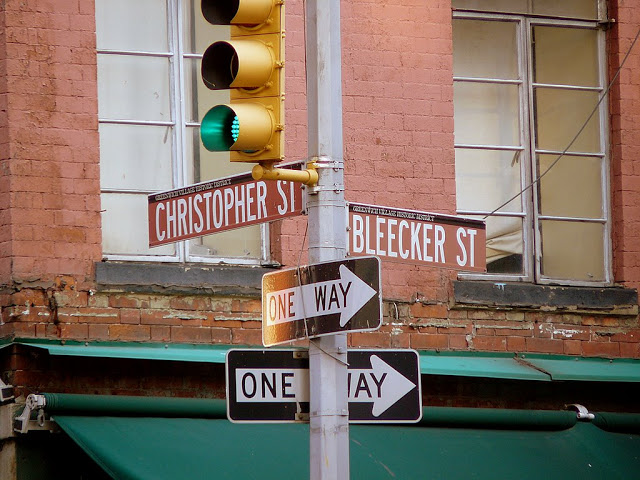The image captures a detailed side view of a street pole laden with various street signs against the backdrop of an aged brick building. The brick building, showing signs of wear with faded, cracked bricks and visible white mortar, features two windows, each with white frames and divided into four panes. Below the windows, a green awning stretches across part of the building.

At the forefront, a gray pole holds multiple street signs and a traffic light. The traffic light, with a yellow frame, shows a green light illuminated. Ascending the pole, a black and white "One Way" sign points to the right, with another identical sign directly behind it, partially obscured but also pointing right. Above these, a reddish-brown sign with white letters reads "Bleecker Street." Further up, another matching sign indicates "Christopher Street."

This intricate composition of signs, light, and architecture conveys a layered, almost bustling intersection scene steeped in both directional cues and architectural character.